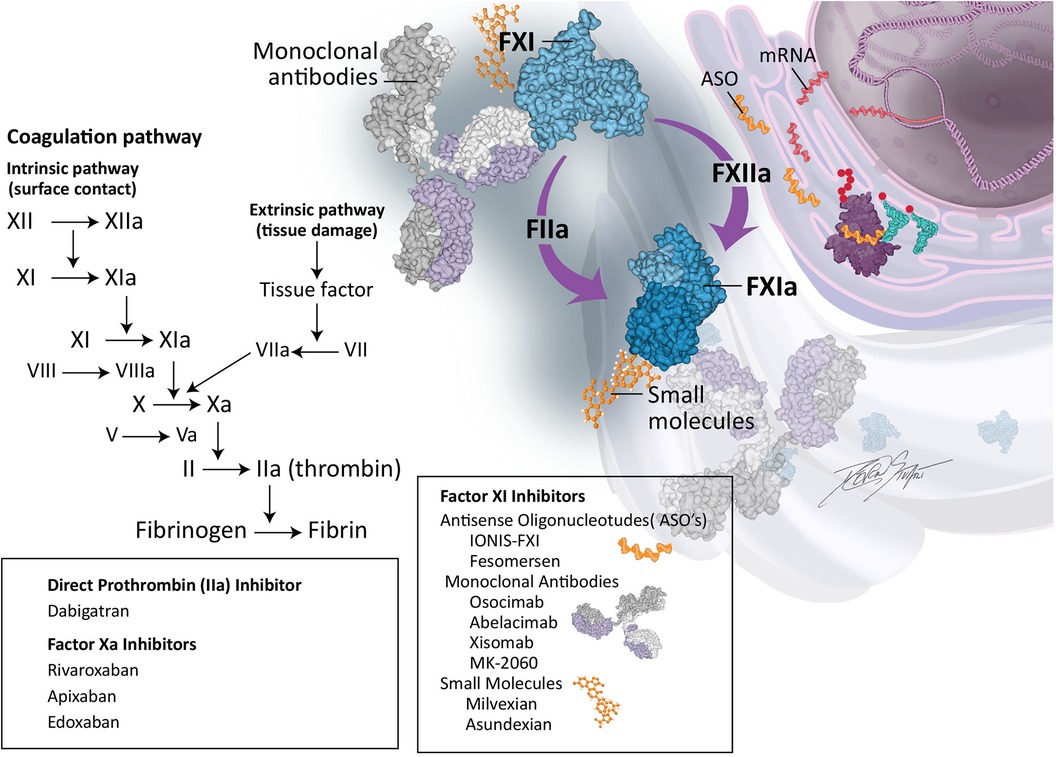The image is a highly detailed and color-coded diagram of the Coagulation Pathway, showcasing both the intrinsic and extrinsic pathways. In the top left corner, it features the text “Coagulation Pathway, Intrinsic Pathway, Surface Contact.” The pathways are illustrated through a series of arrows connecting various Roman numeral-labeled factors (e.g., FXI, FIIA, FXIIA, FXIA) and leading to the formation of fibrin, the material in blood clots. At the bottom, a chart lists different types of inhibitors, including Direct Thrombin Inhibitors (Dabigatrin) and Factor XA Inhibitors (Rivaroxaban, Apixaban, Edoxaban).

On the right side, there's a computer-generated graphic that vividly portrays cells and molecules interacting as per the pathways. This portion includes detailed imagery of DNA being transcribed into mRNA, with proteins such as FX2A being synthesized. The proteins interact with monoclonal antibodies and bind with small molecules. The cells and molecules are depicted in various colors – mainly yellow, red, and lavender – to distinguish their types and functions. Additional diagrams in the top right corner label elements like mRNA and ASO, assisting in the explanation of molecular interactions reflective of the chart on the left. The visual elements, reminiscent of a science textbook page, combine to provide an in-depth educational illustration of blood clotting mechanisms.